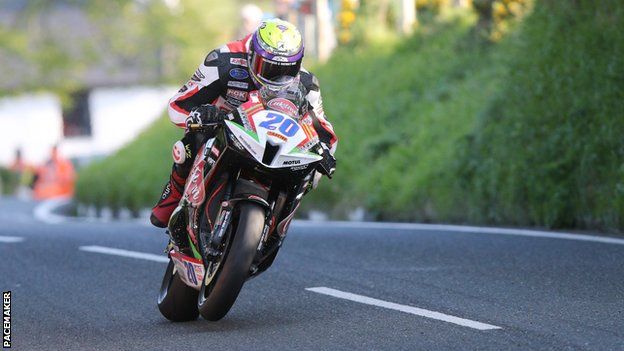This detailed photograph captures a motorcyclist racing along a two-lane highway with a dark asphalt surface and white striped lines. The motorcyclist, dressed in a jacket covered with various sponsor decals in multiple colors, is depicted leaning slightly to the right while balancing by shifting his body to the left. The jacket is predominantly black with wide white stripes down the sleeves edged in red, further adorned with numerous logos. His black gloves with white edges grip the handlebars firmly.

The motorcyclist's helmet is strikingly noticeable with a neon green crown, a purple ring just above the black visor, and blue edging around the visor. His right knee features a white smiley face pad, and his boots or shoes are dark red with black soles.

The sleek, sponsor-covered motorcycle itself is a mix of white and red with the number 20 displayed prominently on the front shield. The motorcycle's front wheel, slightly slimmer than the very wide back wheel, is momentarily off the ground, indicating speed and motion. Both tires appear exceptionally smooth, designed for high performance.

Surrounding the roadway, lush greenery lines the edges, and a steep grassy embankment is visible to one side. In the background, a white building with a roof and a single window further contextualizes the scene. The front of the motorcycle faces toward the camera, leaning slightly, capturing the dynamic energy of the race. Notably, the word "Pacemaker" appears vertically in the bottom left corner of the image.